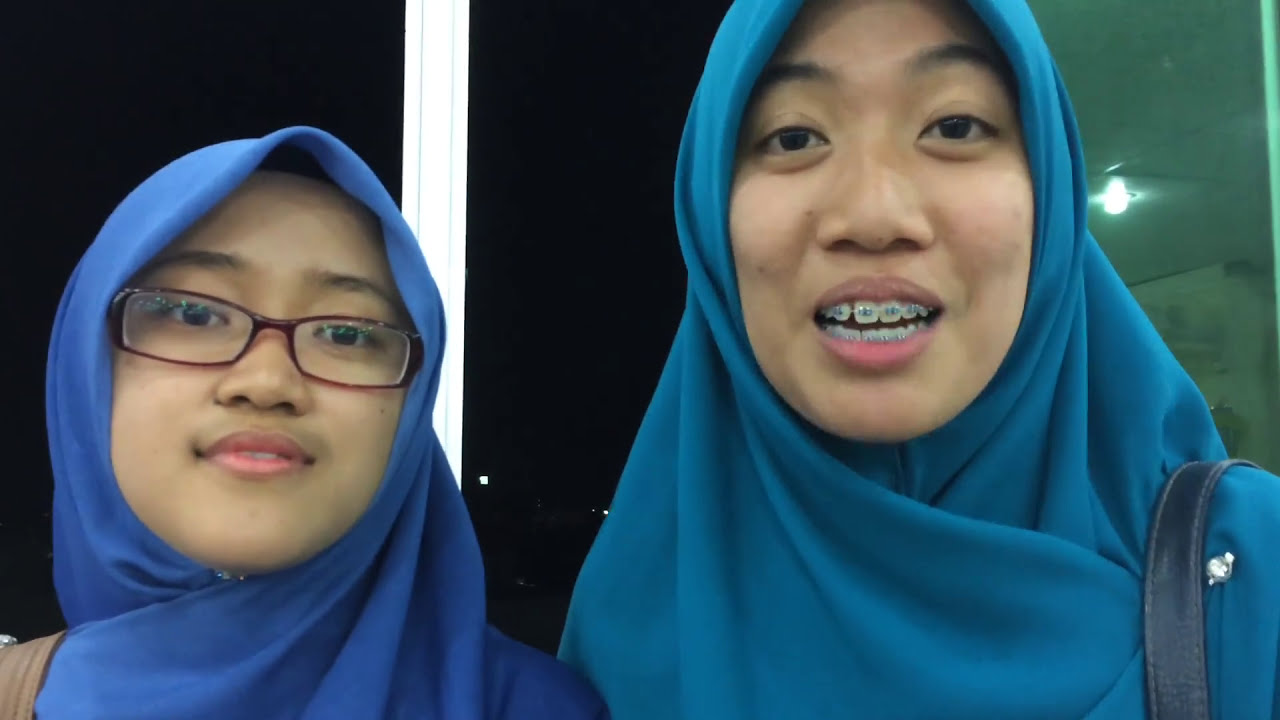The photograph captures two women of Middle Eastern or Asian descent. Both are adorned in traditional head coverings; the woman on the right wears a medium blue burka, and the younger woman on the left sports a darker blue head covering. The woman on the right has a broad, expansive face with almond-shaped eyes, a wide nose, and is distinctly noticeable because she is smiling slightly and wearing braces on her teeth. She also carries a blue purse strap over her shoulder. The younger woman to her left, who appears slightly shorter and has a smaller head, wears rectangular maroon glasses and has a light brown purse strap. They both have gentle smiles on their faces. The background is mostly dark, possibly indicating nighttime, with a bare light bulb hanging from the ceiling and a greenish tint on the side, hinting at the presence of a white structure or house. The overall composition focuses on the women looking directly at the photographer, making it an engaging and vivid portrait.